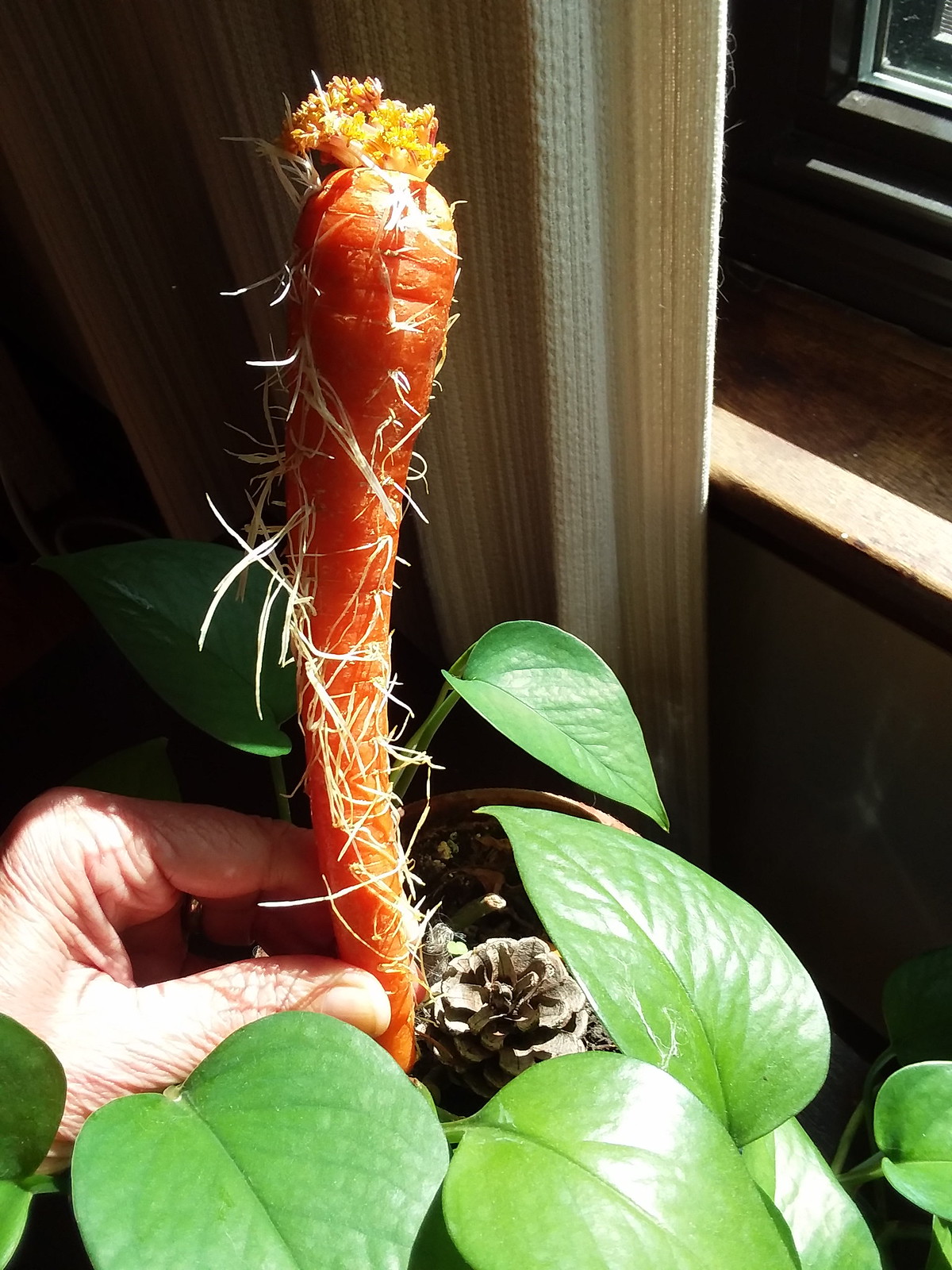The photograph captures a vivid image of a man’s hand, likely belonging to an older individual given the pale, wrinkled skin, holding up a homegrown carrot above a potted plant. The carrot, bathed in sunlight filtering through a beige, woven curtain on the left, exhibits a brilliantly bright orange hue adorned with numerous white, stringy roots that give it a hairy appearance. At the top of the carrot, the foliage has been trimmed down to small yellow stubs. The pot below contains lush, shiny green leaves, and a randomly placed pine cone can be seen among them. The scene is set against a backdrop featuring a glimpse of a window and the soothing glow of natural light, creating a high-contrast, high-quality image that highlights the organic textures and vibrant colors of the subject.